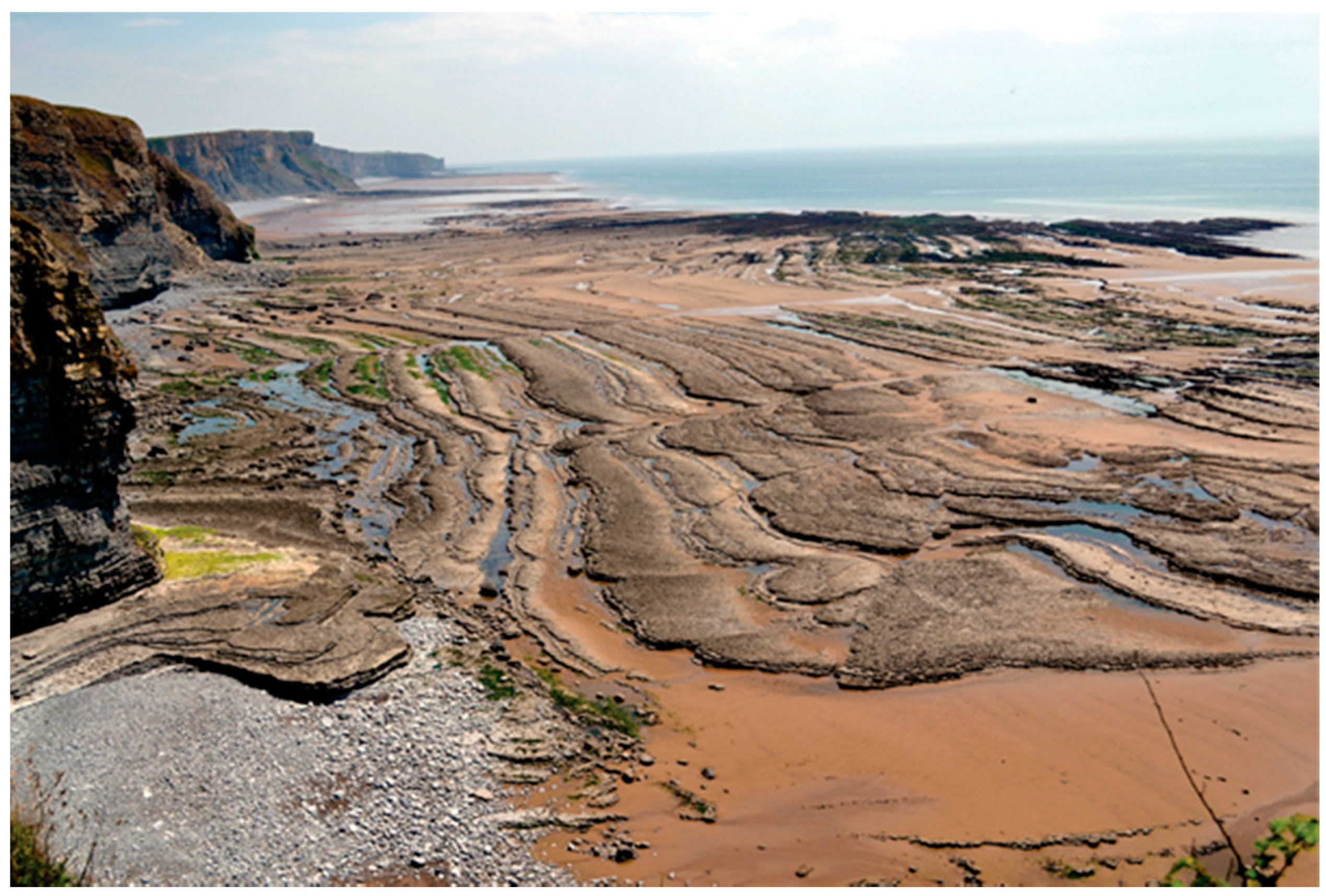This photograph, likely taken from a drone or high vantage point, captures a stunning beach scene with an estuarine or tidal landscape along the ocean. Dominating the left side of the image are steep cliffs, composed of striking brown or reddish-brown rock, stretching upwards and creating an impressive natural barrier. At the base of these cliffs, the rocky terrain transitions into a sandy and muddy expanse on the right side, suggestive of a low tide setting where the ocean has retreated, revealing pools and puddles of water amidst the sand.

The color palette of the scene is rich and varied: the sand is predominantly brown, interspersed with hints of green shrubbery, while the water and the sky above are vivid shades of blue, with the sky featuring scattered white clouds. The cliffs themselves, with their seemingly volcanic origins, add a dramatic touch to the landscape, appearing as if ancient lava flows have repeatedly solidified to form a rugged, yet beautiful shoreline. The image as a whole captures the raw and intricate beauty of this coastal region, from the detailed textures of the rocky cliffs and sandy stretches to the serene blues of the ocean and sky above.